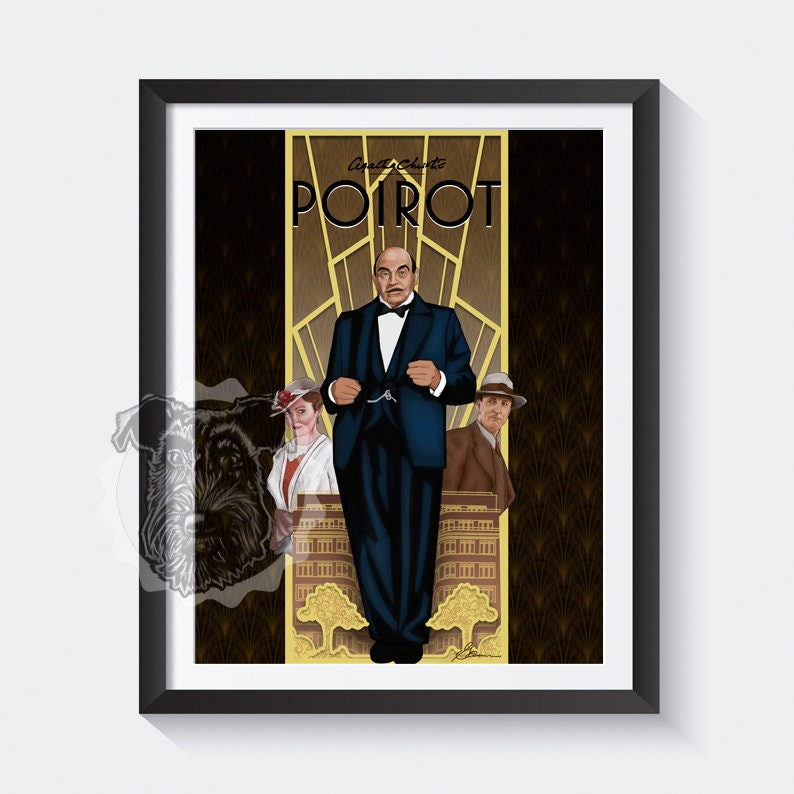This image is a perfectly square framed artwork with a white background. Central to the image is a drawing or painting bordered by a black frame and white matting, flanked by black bars on either side. In the center of the artwork is a gold and brown scene depicting a building and some trees. At the top, there's cursive black text that is difficult to read, followed by "POIROT" in large, all-caps letters. 

Dominating the center is a bald Caucasian man with a mustache and thick eyebrows, dressed in a dark navy suit and black bow tie. He stands formally, hands in an upright position, gazing forward. To his left, a Caucasian woman with a white jacket, white hat featuring a red flower, and red undershirt is visible chest-up. To his right is another Caucasian man in a gray hat and brown suit. Notably, a blurred dog-faced watermark appears on the left side of the image. The overall setting and style suggest that this might be an advertisement or a poster, possibly for an old movie or artistic homage.